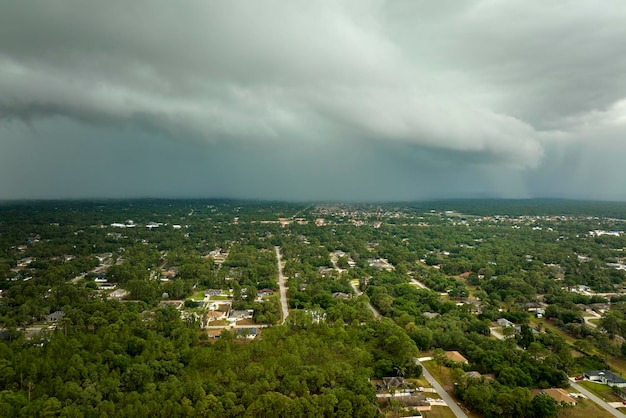This aerial photograph captures a vast, predominantly green landscape, likely a small town enveloped by dense clusters of trees. The foreground highlights sparsely scattered residences with large yards and overall, there are no high-rise buildings, suggesting a predominantly low-rise, ranch-style neighborhood. In the lower left corner, a thick aggregation of trees lacks walkways or clearings, contrasting with the sporadically placed homes just above it. Dominating the skyline are extensive, dramatic storm clouds, creating a dark gray, overcast atmosphere with hints of rain in the far distance, which adds a dynamic, almost melancholic touch to the scene. The horizon is adorned with bluish hills, possibly tinted by the lighting and the encroaching storm. The town itself appears organized in a grid-like fashion with streets interspersing the abundant greenery. The overall terrain is remarkably flat, deepening the sense of a serene, spread-out small town under a looming sky.